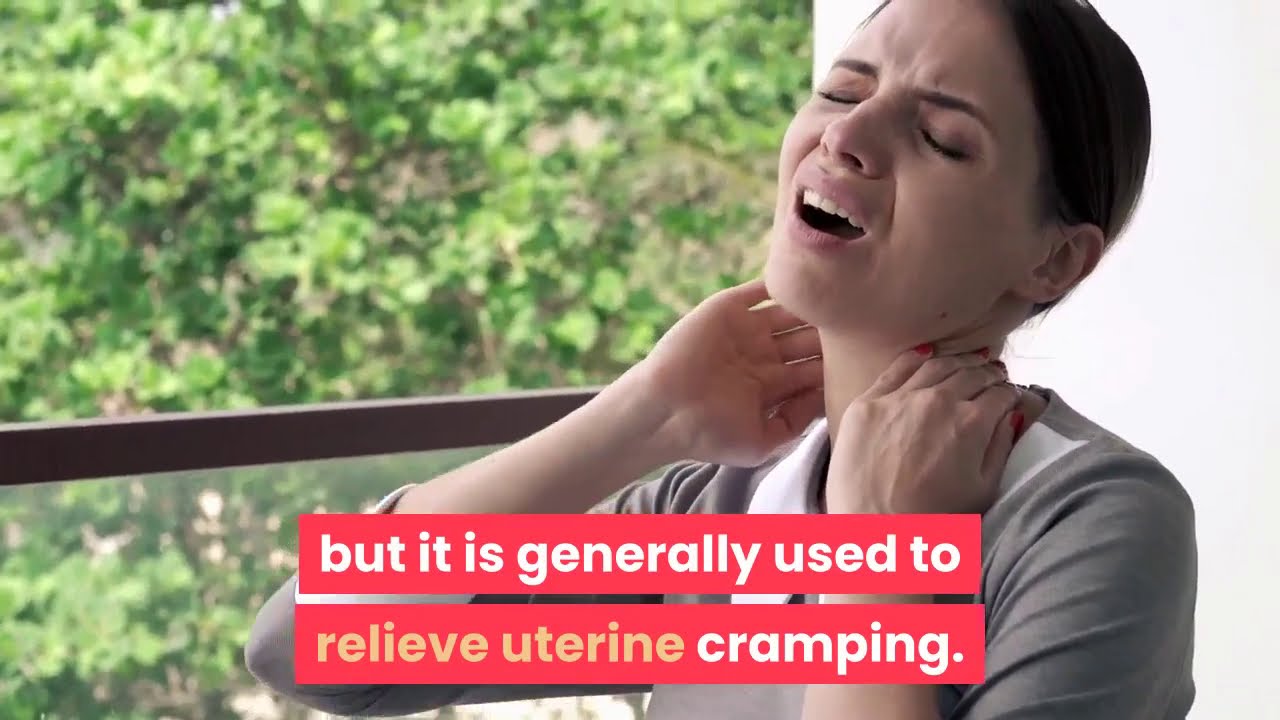The image depicts a woman with brown hair styled in a bun, wearing a gray shirt, positioned on the right side of the frame. She appears to be in significant discomfort, tilting her head back with her eyes closed, her mouth slightly open showing the upper portion of her teeth, and both hands clasped around her neck. Her facial expression is one of pain, with a scrunched upper face and slightly visible red nail polish. Behind her to the left, there's a large window with a brown bar through which one can see a daytime outdoor scene featuring lush green trees with some brown leaves. At the bottom of the image, there's text overlay on a red background stating, "but it is generally used to relieve uterine cramping," with "relieve uterine" highlighted in yellow and the rest of the text in white. The setting appears to be indoors, utilizing natural light from the window, possibly suggesting that this is an advertisement for a pain relief product.